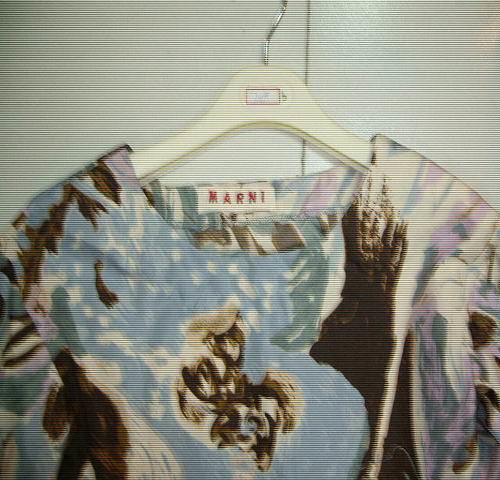This image showcases a shirt on a white hanger with a metal hook, positioned against a white wall that may have horizontal lines due to the photograph's effect. The image has a grainy, CRT filter that gives it a vintage, textured appearance. The shirt features an abstract, tie-dye-like design with light blue as the dominant color, accented by wisps and swirls of brown, purple, and teal. At the center of the shirt appears to be a mythical creature. The collar of the shirt bears a tag labeled 'Marnie.'